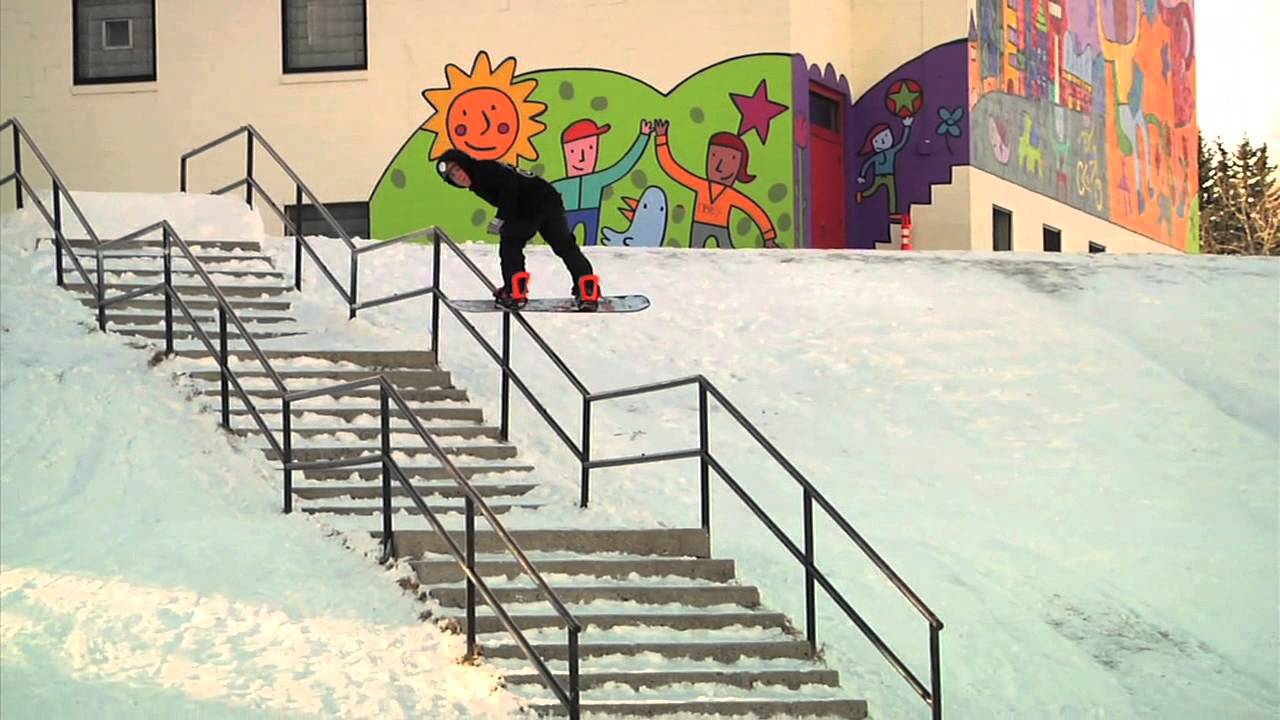This horizontally aligned photograph captures a vibrant and dynamic scene dominated by a large mural on the right side, possibly painted on the side of a school building. The sky is pale, with an almost white hue tinged with yellow at the edges, suggesting bright sunlight. Coniferous or pine trees, triangular in shape, are visible in the upper right part of the image.

The mural itself is a burst of colors and activity. On the right side of the mural, a woman or girl with long black hair, dressed in a yellow shirt, appears to be sitting in a green chair with her arms upwards. At her feet are multicolored objects, possibly toys, and a pink and peach polka-dotted creature with a pointy snout smiles nearby.

To the left of this, a cityscape extends from left to right, featuring pink, blue, green, and yellow buildings, along with a red stop sign. Below the cityscape, a child in green pants and a blue long-sleeved shirt plays with an orange and green starred ball. A flower sits to the right of the child, and further along, a red door with a window at its top is part of the mural, angled within a corner of the building.

The mural also includes various playful elements: stairs drawn in a cubist style with a purple background, a light blue duck with an orange beak, and two kids high-fiving—an African-American girl with dark hair in an orange shirt and gray pants, and a white boy in a red hat and teal shirt with blue pants. The dynamic scene is completed by patches of green hills, a smiling orange and yellow sun, and a magenta star above the girl's head.

In front of the building and mural is a snowy, sculpted-looking hill. A set of gray cement staircases with three landings and horizontally barred railings descends diagonally from the left. In the middle of this slope, a Caucasian male snowboarder in black attire with orange bindings is grinding down the rail backward. His snowboard, partially positioned on the rail, shows an indistinct pattern, while his hooded head, tilted towards the viewer, reveals a white forehead band. The overall scene is energetic and visually rich, combining artistry with the thrill of snowboarding.